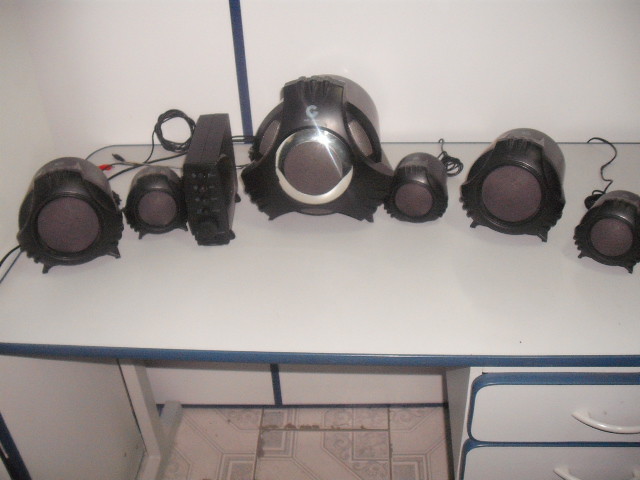In this realistic, horizontally-oriented photograph, an indoor scene is depicted. The background comprises a white wall that features a vertical blue stripe on the left side. The floor appears to be covered with white linoleum tiles adorned with a subtle grayish-blue pattern. Central to the image is a white desk, which stands prominently. The desk boasts a white surface and blue trim, with a cabinet containing at least two visible drawers, each accented with white pull knobs and blue trim. The open space beneath the desk is designed for seating, while on the right side rests the aforementioned drawers and cabinet.

On top of the desk is an array of electronic equipment, predominantly black in color. This equipment includes approximately six round speakers of varying sizes, organized by three distinct dimensions: three small, two medium, and one larger speaker. In addition to the speakers, there is a rectangular device, likely an internet modem. The largest round device, positioned centrally on the desk, features a triangular front and a prominent white letter 'C'. The round devices vary in size, with the smallest one being a bit larger than a baseball and the largest one slightly bigger than a basketball. Numerous black cables are visible, connecting the various electronic pieces, with their screens facing outward towards the viewer.